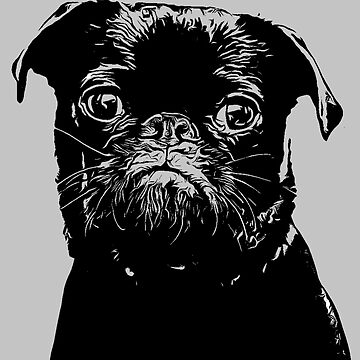The image is a meticulously detailed black and white photograph of a small dog, specifically a Brussels Griffon, although it bears a resemblance to a pug in its features. The background is a plain light gray, accentuating the dog without distractions. The central focus is the dog's face, depicted from the top of its head down to about mid-neck. The photograph utilizes contour filters to enhance contrast, resulting in notable white highlights on the edges of the floppy ears, stubby nose, and around the mouth, adding depth to the otherwise dark facial features. The dog's expression is somber, with large, round eyes that appear to have floating objects in them due to the high contrast effect. The painting captures the essence of the dog's features with flattened forward ears and a pronounced frown, creating a stark, visually striking portrait without any text or additional elements. The square framing of the image further isolates the dog, enhancing the simplicity and intensity of the piece.